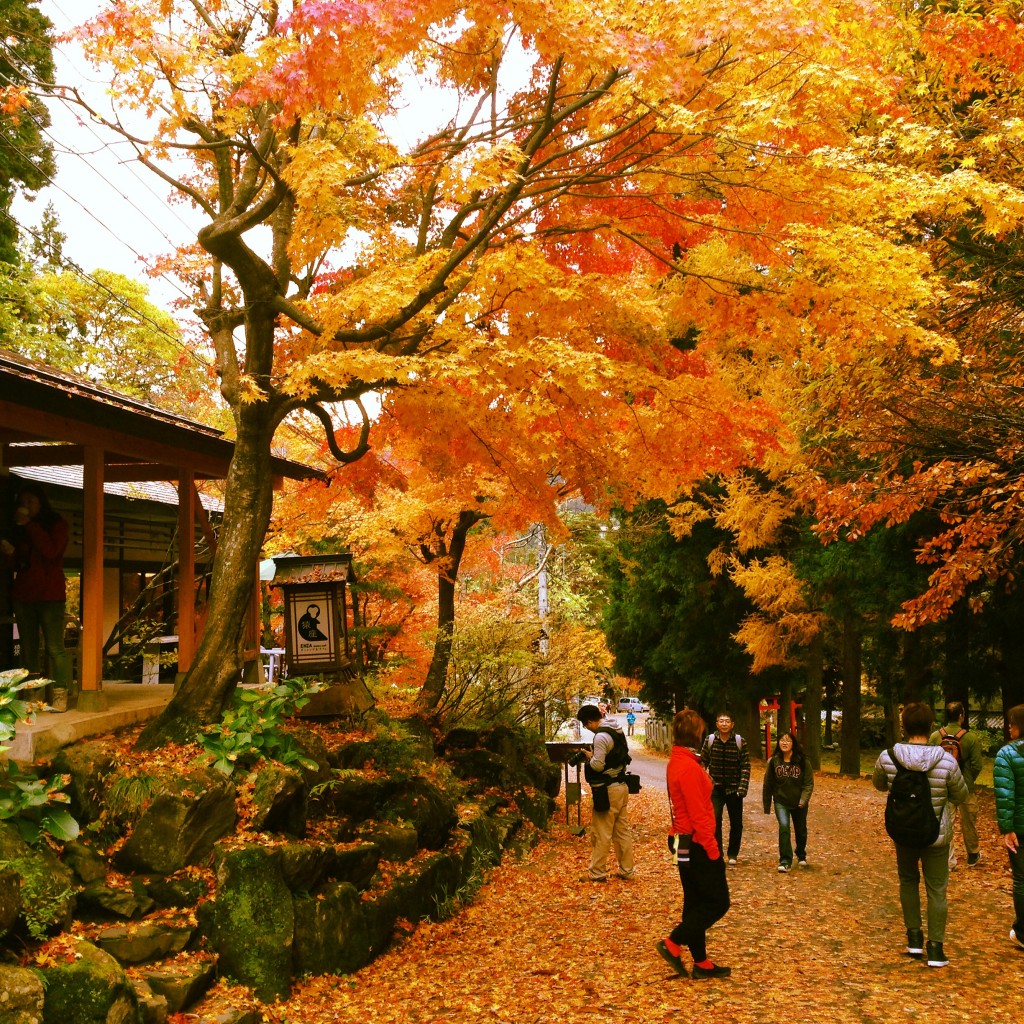The photograph captures a vibrant autumn day in a park, showcasing an explosion of fall colors with red, orange, and yellow leaves dominating the scene. The main focus is a wide path or sidewalk, covered in a carpet of fallen orange and yellow leaves, creating a vividly colorful landscape. This path is bordered on the left by a stunningly bright deciduous tree with blazing orange and yellow foliage that overhangs the walkway and on the right by greener coniferous trees. Along the path, a total of seven people can be seen, some walking away and others towards the camera, with a noticeable few carrying backpacks and wearing winter coats, including a silver and blue one and a green outfit with an orange backpack. In the lower left corner, a stone wall is partially visible, adorned with the same vibrant fallen leaves. Directly behind the tree to the left, there's a distinctive building resembling a pagoda, stage, or porch, with beams supporting its structure and electricity wires above. Near this building, there's an informational sign, which intriguingly features a drawing of a monkey. The entire scene is beautifully captured, emphasizing the sheer brilliance of the autumnal colors and the bustling activity of people enjoying the park.